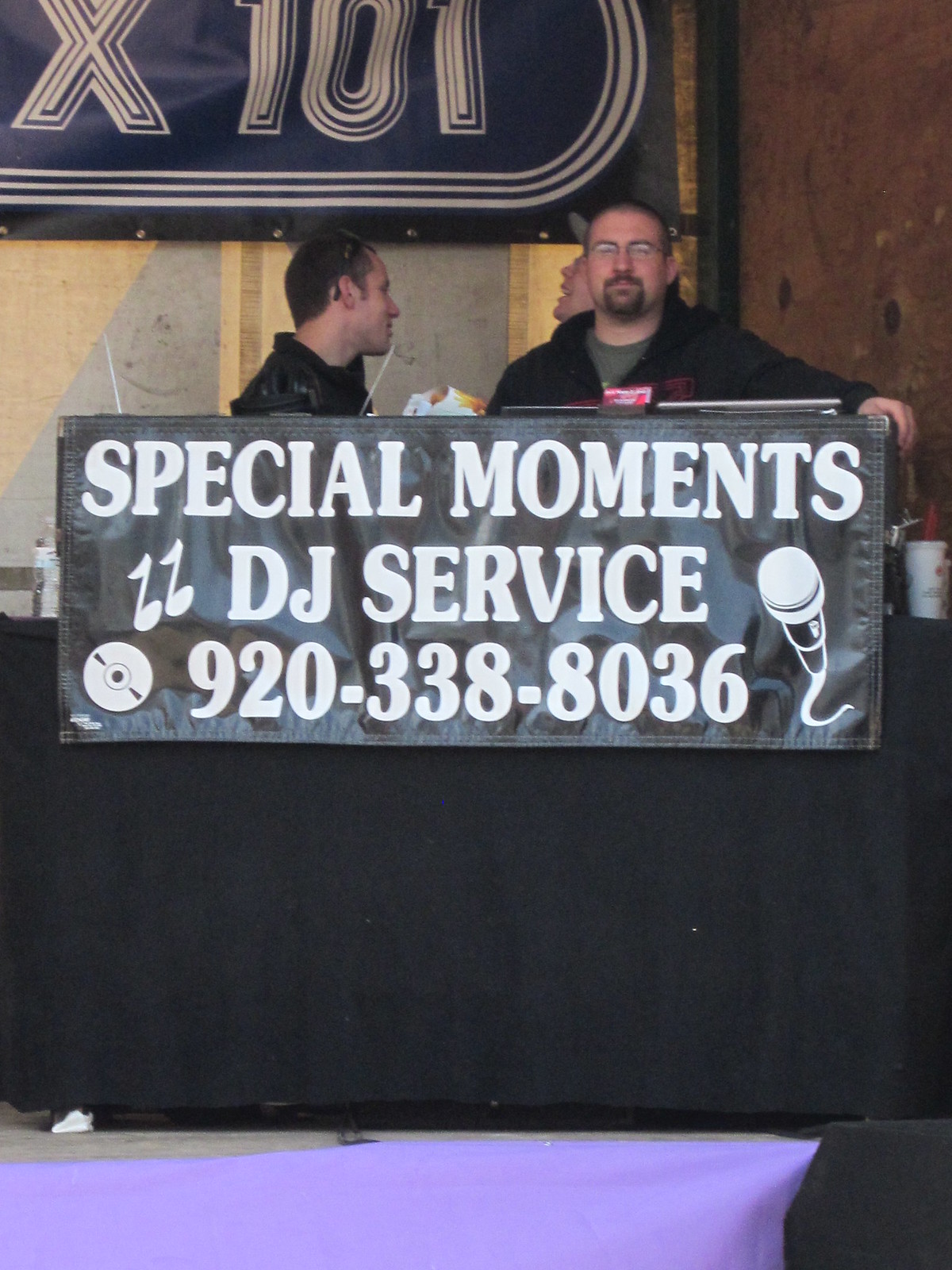This photograph captures a lively scene featuring three men, likely DJs, at what seems to be a promotional event for a DJ service. Positioned prominently at the center of the image is a black podium bearing a sign that reads "Special Moments DJ Service" along with the contact number "920-338-8036" in uppercase white letters. Decorating the sign is a white CD located in the lower left corner and a black and white microphone on the right.

On the left side of the image stands a man in a black jacket engaged in animated conversation with another man situated behind the podium. This second man, possibly singing, has his mouth open and eyes closed, adding a dynamic element to the scene. In front of him is the third man, sporting a black jacket over a green t-shirt and wearing eyeglasses, who is directly looking at the camera.

The overall setting suggests that they are either hosting a DJ session, participating in a DJ convention, or presenting their DJ services at a radio station event, as indicated by the possible presence of a radio sign in the background. The detailed elements of the microphone and CD contribute to the event's professional and musical atmosphere.